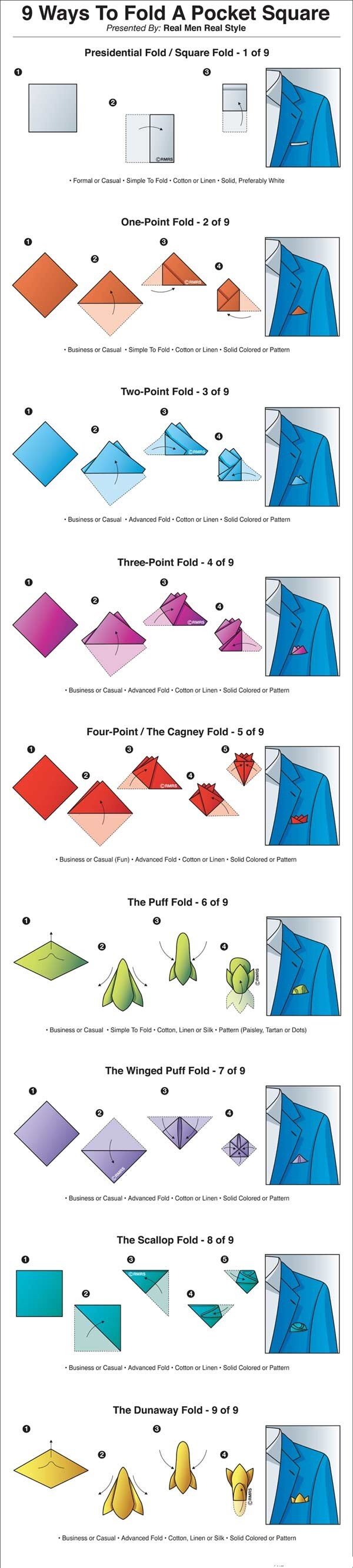This detailed and colorful illustration titled "Nine Ways to Fold a Pocket Square" by Real Men Real Style showcases nine distinct techniques for folding a pocket square. Each method is illustrated with a step-by-step guide positioned on the left and a visual of the final look inserted into a man’s jacket pocket on the right. The folds demonstrated include the presidential fold, one-point fold, two-point fold, three-point fold, four-point fold, a puff fold, a wing puffed fold, a scallop fold, and a dunaway fold. The instructions are rendered in various vibrant colors—white, brown, blue, purple, reddish rust, green, lilac, aqua, and gold—making the learning process visually engaging. The headline in black text at the top underscores the theme of the image. The entire arrangement is presented in a portrait orientation and is a blend of illustration with descriptive text, effectively guiding viewers through each folding sequence.